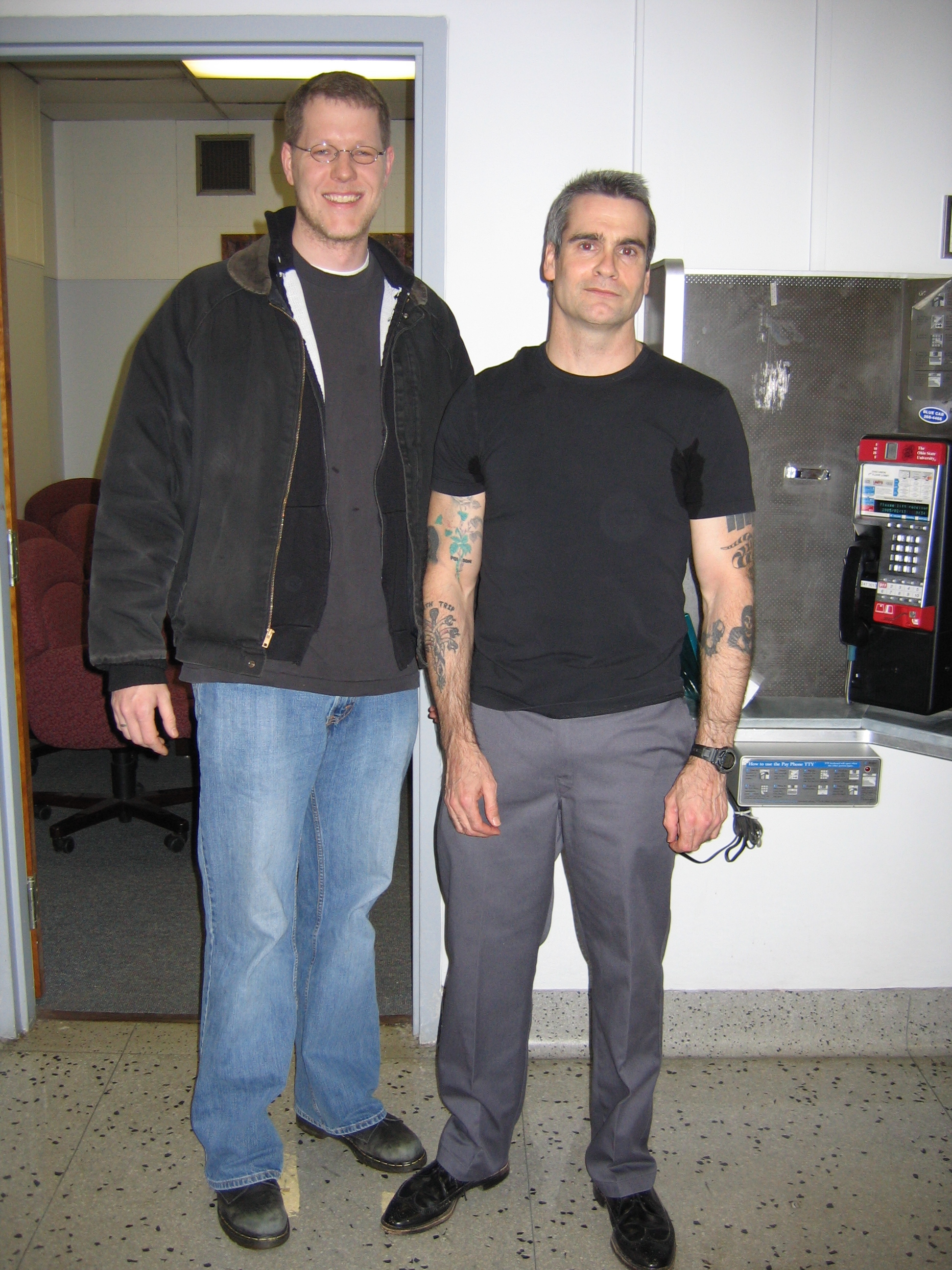In the photograph, two men are standing side by side, smiling at the camera. The man on the left, a tall white male with dark hair, wears eyeglasses, jeans, black boots, a gray t-shirt, and a black jacket which might be layered. The man on the right, who appears to be a singer, is a white male with black hair tinged with gray. He is dressed in a black t-shirt, gray slacks, and black shoes, accessorized with a black watch on his left wrist and visible tattoos on his arms. Behind them, slightly to the right of the singer, is a payphone with a silver casing. Additional background elements include ceiling lights, tiles on the floor, a couple of chairs past a doorway on the left, and vents up top towards the middle left. The photograph features a mix of colors such as black, gray, white, beige, burgundy, green-blue, silver, and brown, suggesting it might have been taken some time ago, likely by a fan, given its imperfect quality.